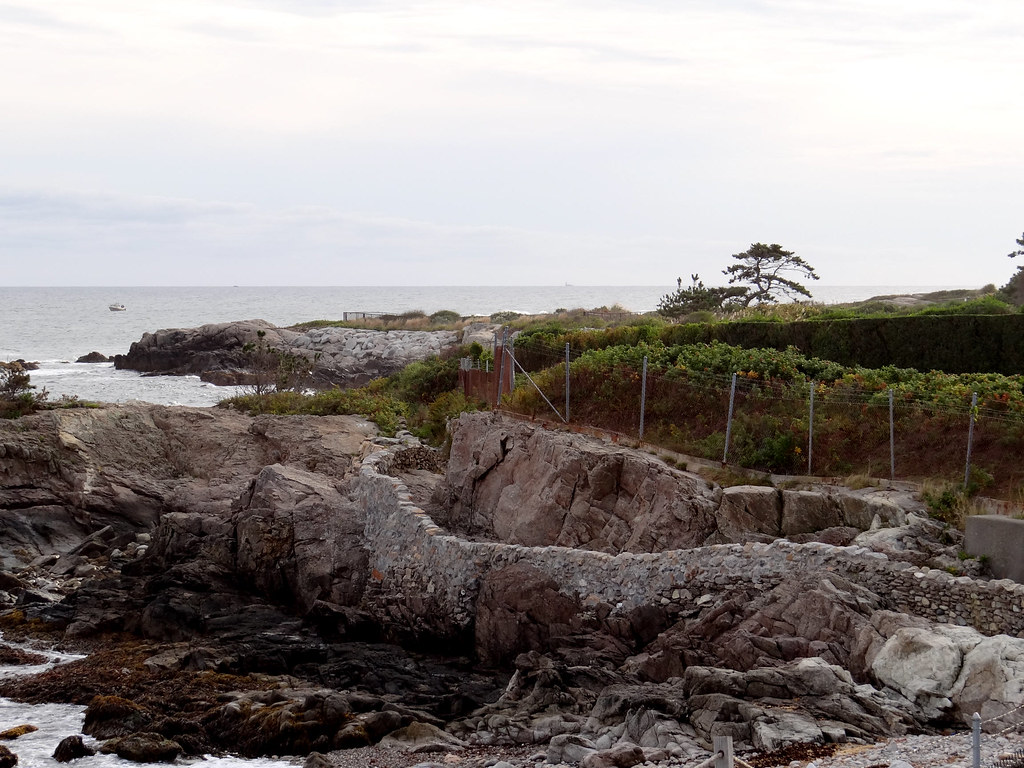The image captures a wide, rectangular photograph of a rocky shoreline meeting a grayish-blue body of water under a mostly cloudy, pale to white sky. The horizon line sits just above the mid-center, slicing horizontally across the image. At the shoreline, a varied collection of rocks dominates the foreground, interspersed with brown seaweed. To the far left, faint waves are visible as they brush against the shore. Mid-image, a steel fence delineates the rocky ground from the shore, enclosing an array of green bushes with small fruits. Further in the background, lanky-branched trees and manicured hedges are visible. On the far right, additional clusters of rocks continue to outline the water. A tiny boat is seen in the distant left, emphasizing the photograph’s broad perspective. The overall scene is bathed in daylight, with the intricate details of the rocky landscape, vegetation, and distant elements clearly depicted.